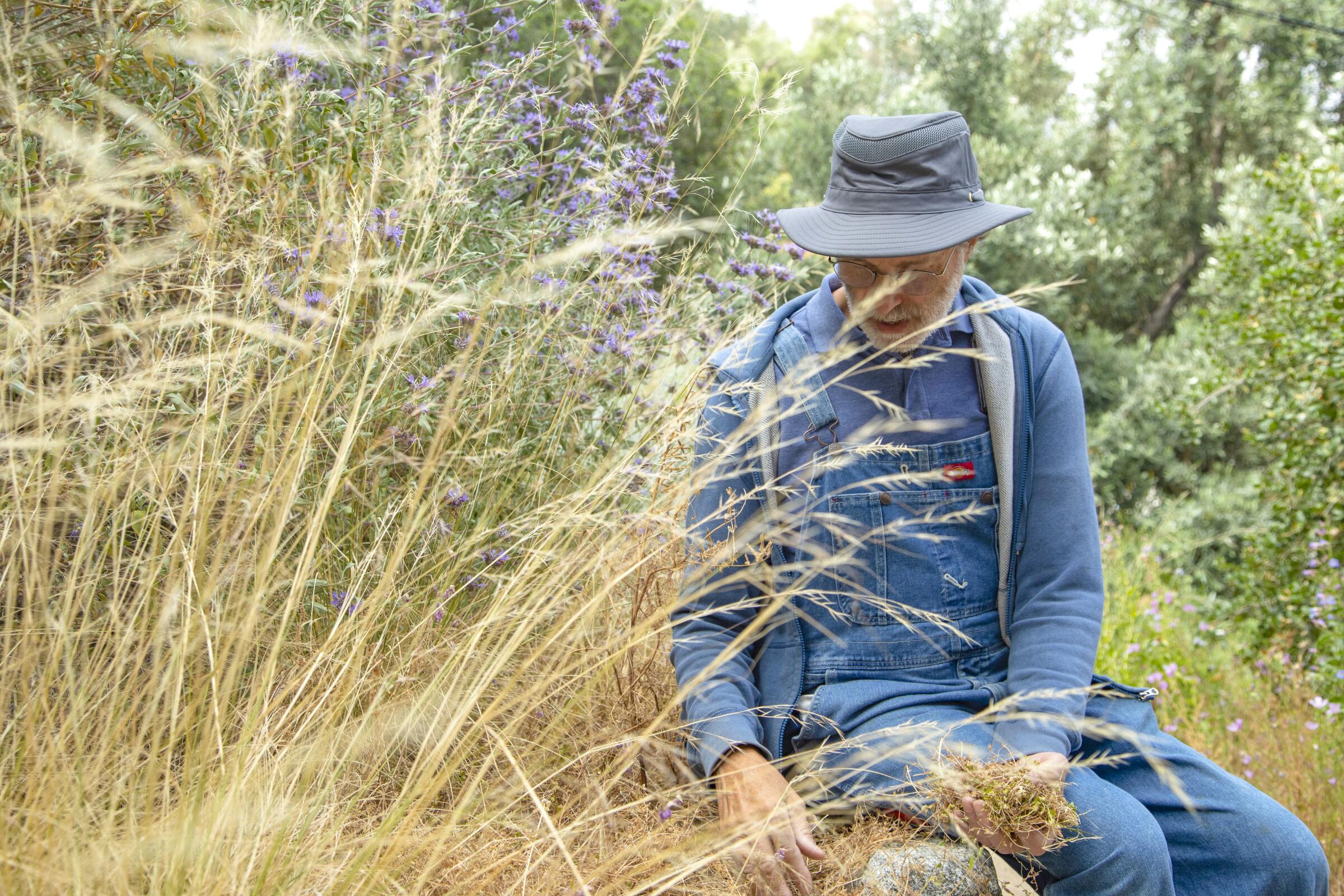The photo features an elderly man sitting in a lush field or garden, surrounded by various types of plant life. To the left of the frame, wispy straw-colored grasses and purple flowers proliferate, creating a vibrant foreground. The man, with glasses and a neatly trimmed gray beard, is wearing blue denim overalls paired with a long-sleeve blue shirt. He has layered his outfit with a blue zip-up sweatshirt and tops it off with a gray cloth cap. He appears to be intently examining the flora around him, his gaze directed downwards. Behind him, green trees and shorter, vibrant grasses form a tranquil background, adding depth to the natural setting. The overall scene evokes a peaceful connection between the man and his environment, possibly suggesting a moment of contemplation or studying the diverse vegetation around him.